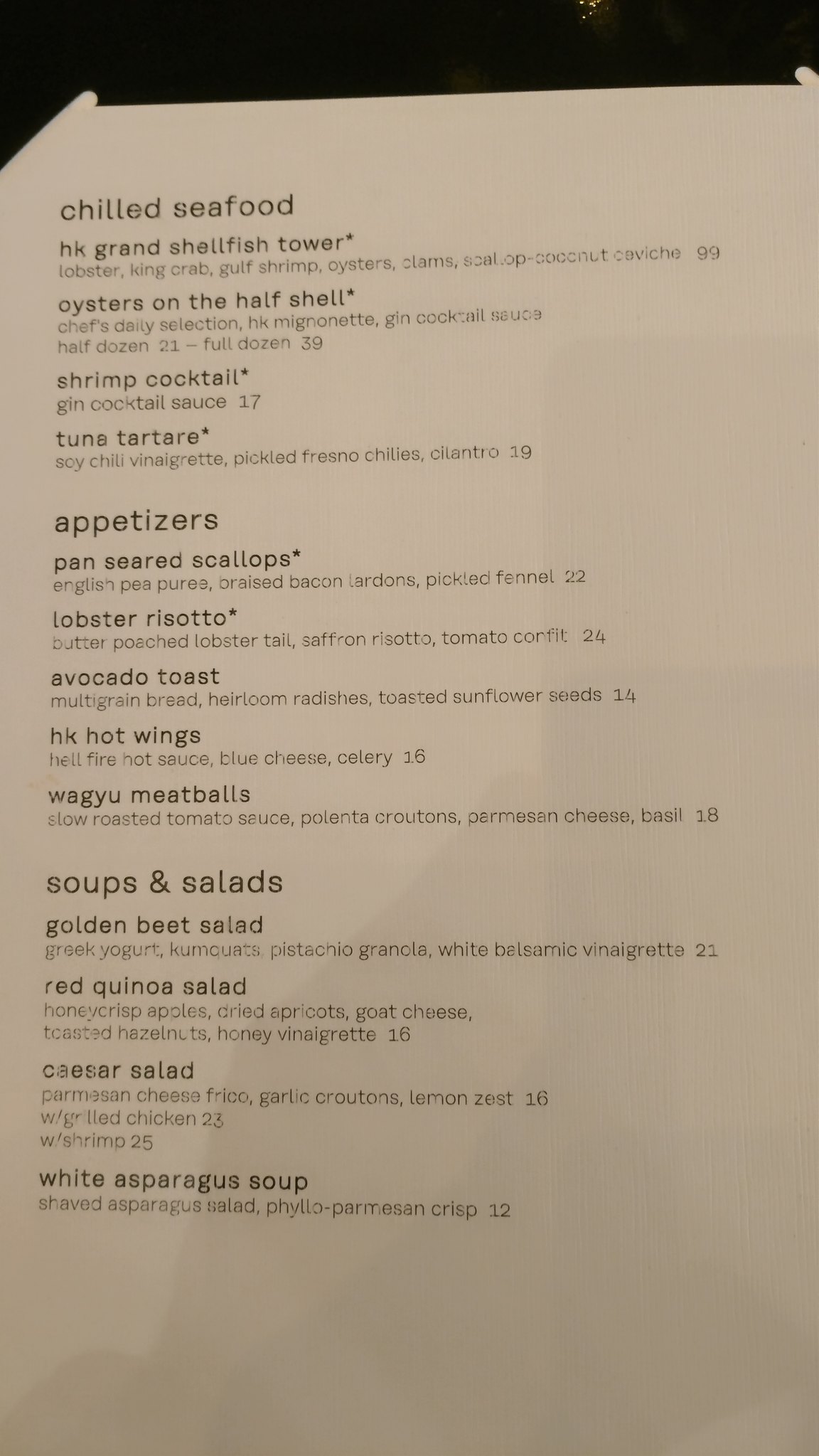This is a photograph of a menu, featuring a tall piece of eggshell white paper with a somewhat rough texture. Slightly light gray shadows appear on the right and bottom edges of the frame, casting from top to bottom. The text on the menu is in solid black.

**Chilled Seafood:**

- **HK Grand Shellfish Tower** (*): Lobster, king crab, Gulf shrimp, oysters, clams, scallop coconut ceviche - $99
- **Oysters on the Half Shell** (*): Chef's daily selection with Hong Kong mignonette and gin cocktail sauce
  - Half dozen - $21
  - Full dozen - $39
- **Shrimp Cocktail** (*): Served with gin cocktail sauce - $17
- **Tuna Tartare** (*): Soy chili vinaigrette, pickled Fresno chilies, cilantro - $19

**Appetizers:**

- **Pan-Seared Scallops** (*): English pea purée, braised bacon lardons, pickled fennel - $22
- **Lobster Risotto** (*): Butter-poached lobster tail, saffron risotto, tomato confit - $24
- **Avocado Toast**: Multigrain bread, heirloom radishes, toasted sunflower seeds - $14
- **HK Hot Wings**: Hellfire hot sauce, blue cheese, celery - $16
- **Wagyu Meatballs**: Slow-roasted tomato sauce, polenta croutons, Parmesan cheese, basil - $18

**Soups and Salads:**

- **Golden Beet Salad**: Greek yogurt, kumquats, pistachio granola, white balsamic vinaigrette - $21
- **Red Quinoa Salad**: Honeycrisp apples, dried apricots, goat cheese, toasted hazelnuts, honey vinaigrette - $16
- **Caesar Salad**: Parmesan cheese frico, garlic croutons, lemon zest
  - With grilled chicken - $23
  - With shrimp - $25
- **White Asparagus Soup**: Shaved asparagus salad, phyllo Parmesan crisp - $12